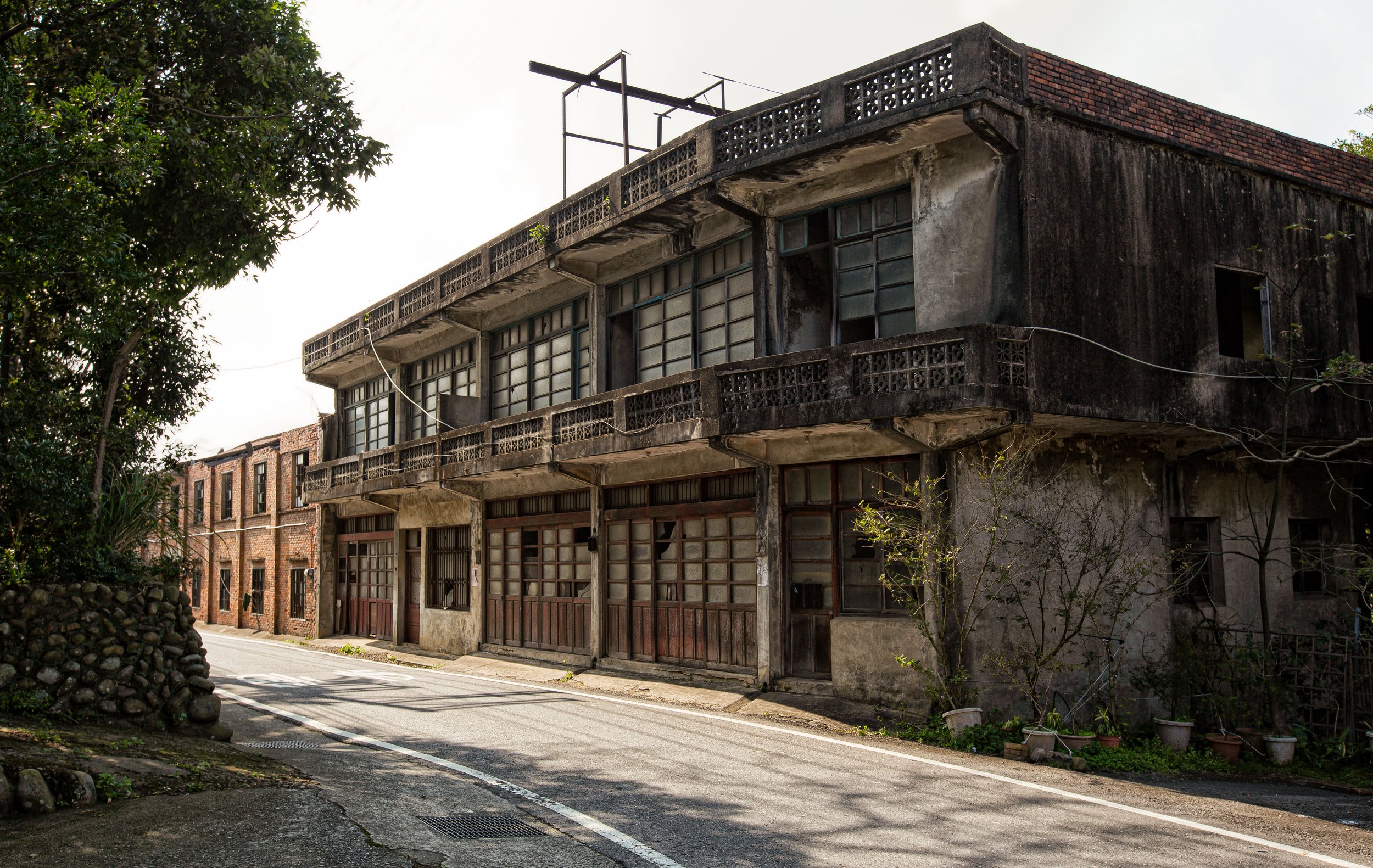This color photograph captures an evidently abandoned, decrepit building with significant external damage. The structure showcases dark, deteriorated walls with substantial water damage, particularly around the upper balcony area, creating a hazardous appearance. The two-story edifice features brown, black-framed windows, many with broken or missing panes, revealing the dark voids within. The building's front sports a porch with a concrete banister above a cluster of dark brown doors. Located directly on an asphalt roadway marked with white lines, the property is surrounded by a barren, lifeless environment. A stone wall with a few sparse trees sits on the opposite side of the road, with potted plants, all in poor health, scattered around the building. The sky overhead is a dreary gray, adding to the overall sense of desolation.